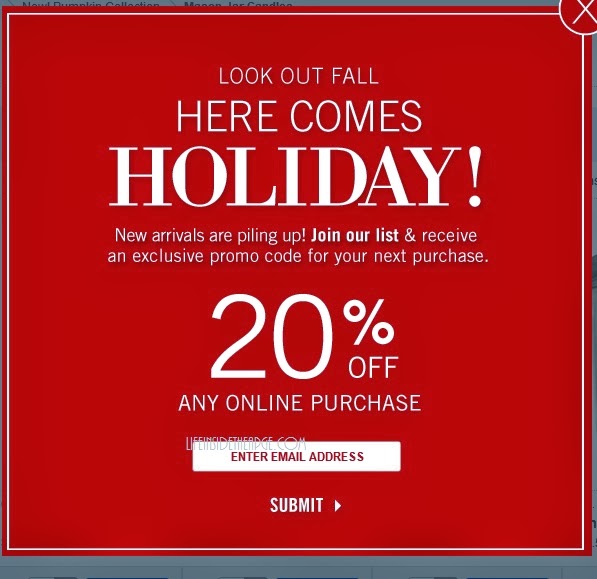The image showcases a vibrant red pop-up coupon commonly seen on retail websites. The coupon has a square shape and features white text on a striking red background. At the top of the coupon, in large, bold font, is the phrase, "Look out fall, here comes holiday!" with an exclamation point emphasizing the excitement. Below this, in smaller text, it reads, "New arrivals are piling up. Join our list and receive an exclusive promo code for your next purchase." Further down, the coupon highlights a special offer: "20% off any online purchase." 

To take advantage of this offer, users are prompted to "Enter email address" followed by a "Submit" button. The overall design is simple yet eye-catching, aimed at encouraging users to subscribe to the mailing list to receive a discount on their next purchase. The repeated phrase, "Look out fall, here comes holiday!" serves to attract attention and emphasize the season's new arrivals and special promotions.